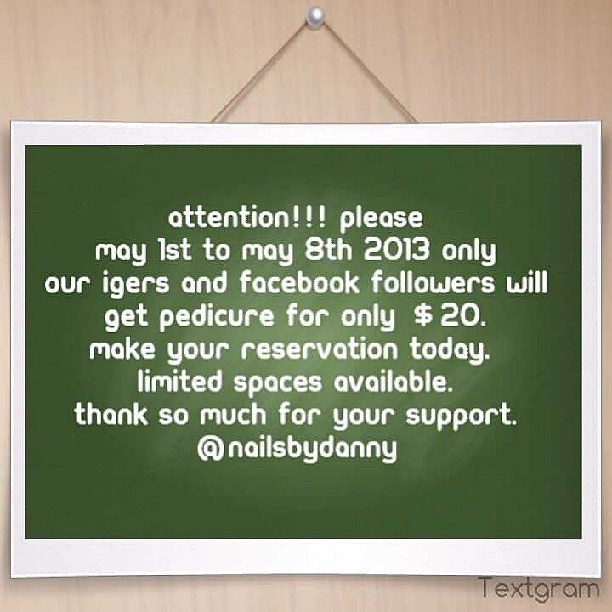In the center of a digital image is a rectangular sign hanging on a light brown, wood-grain wall. The sign is suspended from a silver tack at the top center of the image by a thin triangular string. The sign features a wide white border with a green center that has a gradient effect, becoming lighter towards the center. In bold white font, the sign reads: "Attention!!! Please May 1st to May 8th, 2013 only, our IGers and Facebook followers will get a pedicure for only $20. Make your reservation today. Limited spaces available. Thanks so much for your support, @Nails by Danny." At the very bottom right corner, there is a logo that says "Textgram."